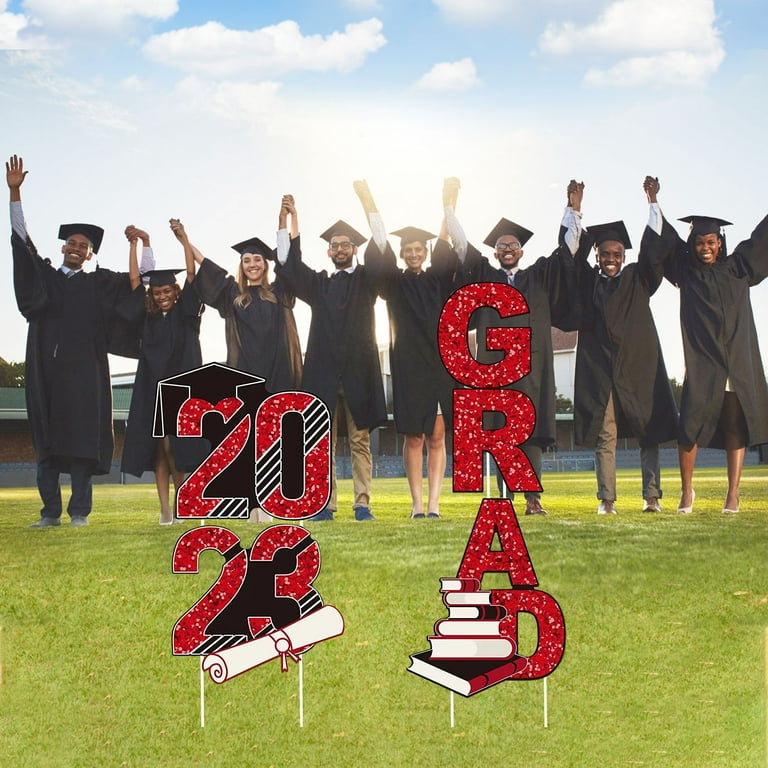In a sunlit field under a vibrant blue sky dotted with fluffy white cumulus clouds, eight high school graduates stand proudly on well-trimmed grass, celebrating their milestone. Wearing black graduation gowns and caps, the group—comprising an even mix of males and females—holds hands and raises them high in a display of unity and joy. The scene is brightened by signs in the background, boldly proclaiming "2023 Grad" in vivid colors of red, yellow, black, and green.